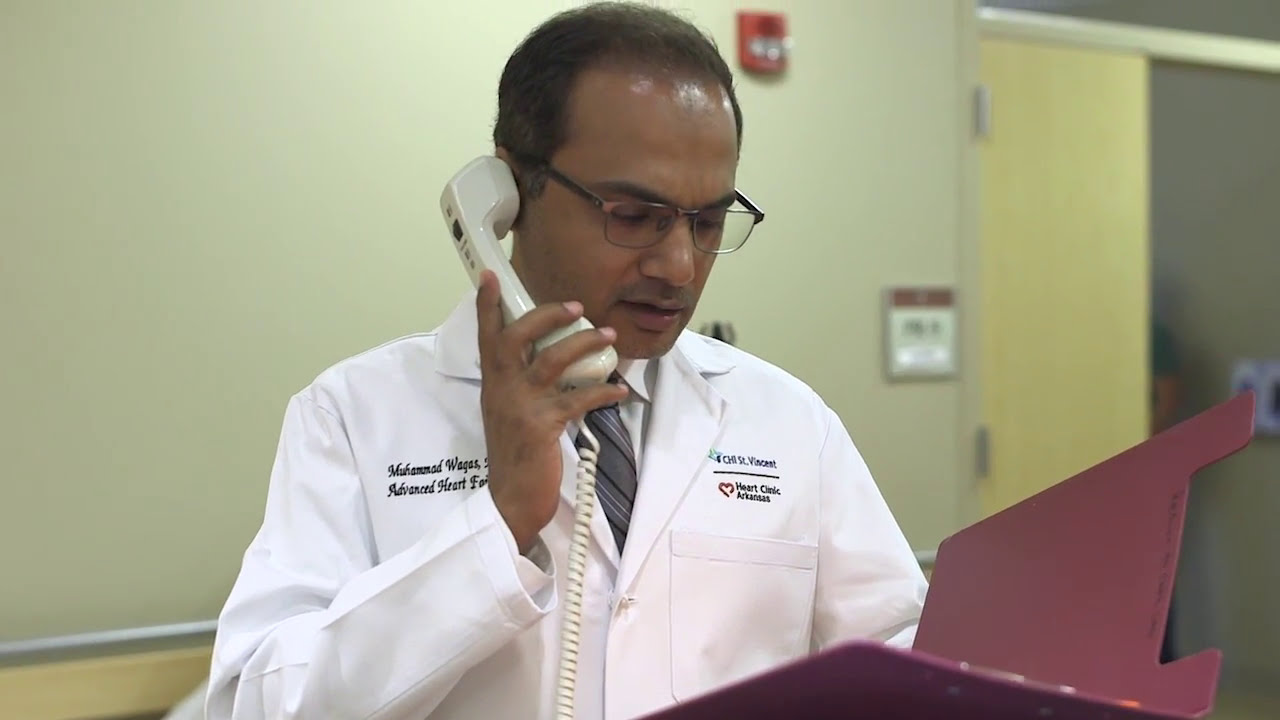The photograph depicts a dark-skinned doctor of Indian ethnicity, with short, neatly combed salt-and-pepper hair, speaking into a phone held up to his right ear while reading from an open maroon (burgundy) medical chart held in his left hand. He is dressed in a white lab coat over a white collared shirt, and a gray tie with black and white stripes. The right breast of his coat bears his name, "Mohammed Weigas," while the left features a logo with a red heart and the text "Heart Clinic, Arkansas" followed by "Advanced Heart." The doctor is wearing glasses and standing in a clinical setting with a light green wall and a wooden door to the right, as well as a red fire alarm and a black and white sign near the door. The overall composition is a horizontal rectangle, roughly twice as wide as it is tall, showing the doctor from his mid-torso up. He appears to be reviewing and possibly dictating patient results, creating a focused and professional atmosphere.